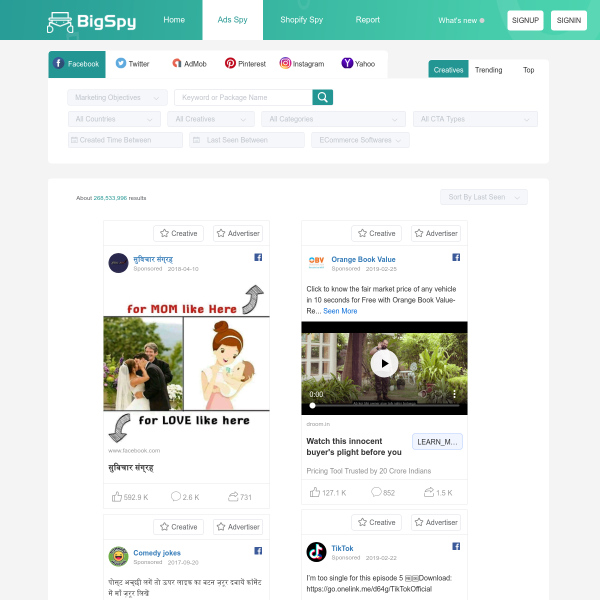The image is a screenshot of the Big Spy website. The top menu is set within a green bar that spans horizontally from left to right, and appears to be center-justified. The menu options listed are: Home, Ad Spy, Shop, Shopify Spy, and Report. The 'Ad Spy' option is currently selected and is highlighted by a white box around it.

Below the top menu, there is another section displaying icons for Facebook, Twitter, Pinterest, Instagram, and Yahoo. The Facebook icon is highlighted with a green box around it, indicating it is selected.

Further down, there are search bars labeled for different purposes: Marketing, Keyword, or Package Name. Additionally, there are seven more text input fields below these search bars.

At the bottom of the screenshot, there is another separate white box containing several items, including a video thumbnail with text that reads, "Watch this innocent buyers - Played before you."